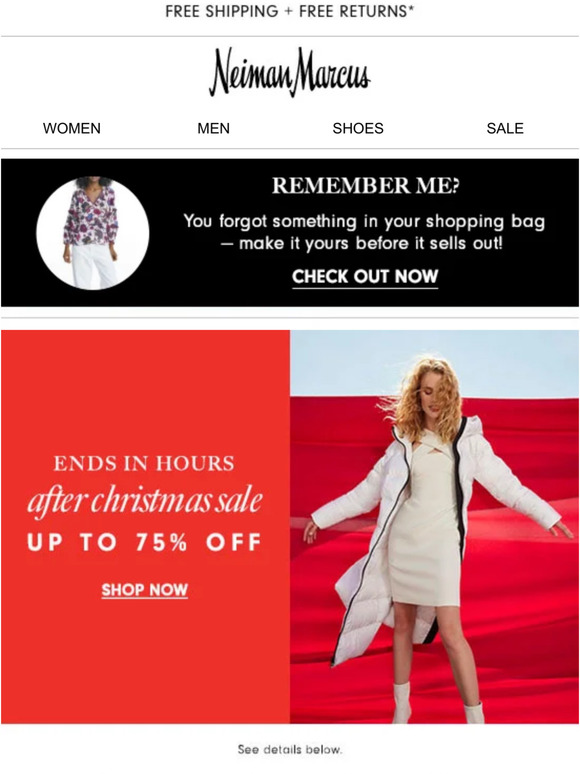This is a detailed screenshot of a shopping website, Neiman Marcus. At the very top, in the middle of the screen, there is a black text announcement: "FREE SHIPPING + FREE RETURNS*". The "+" symbol is used instead of the word "plus" and there is an asterisk next to "returns". Below this text is a thin, horizontal gray line. Following the line, the Neiman Marcus logo is displayed in black cursive text. 

Underneath the logo are tabs categorizing shopping options: "Women," "Men," "Shoes," and "Sale". Beneath these tabs, there is a black rectangle featuring a message in white text: "Remember me? You forgot something in your shopping bag - Make it yours before it sells out. Check it now." The phrase "Check it now" is underlined. To the left of this text, there is an image of an African-American woman dressed in white pants and a floral t-shirt. The image captures her from the chin to her knees, excluding her head and the bottom of her legs.

Further down, there's an advertisement on the left side of the screen. It features a red rectangle with white text reading: "ENDS IN HOURS. After Christmas Sale - Up to 75% Off. Shop Now." The phrase "Shop Now" is underlined, indicating it might be a clickable link. To the right of this text, a Caucasian woman with blonde hair is modeling Neiman Marcus clothing. She is dressed in a white dress and a knee-length white puffer jacket, paired with white boots.